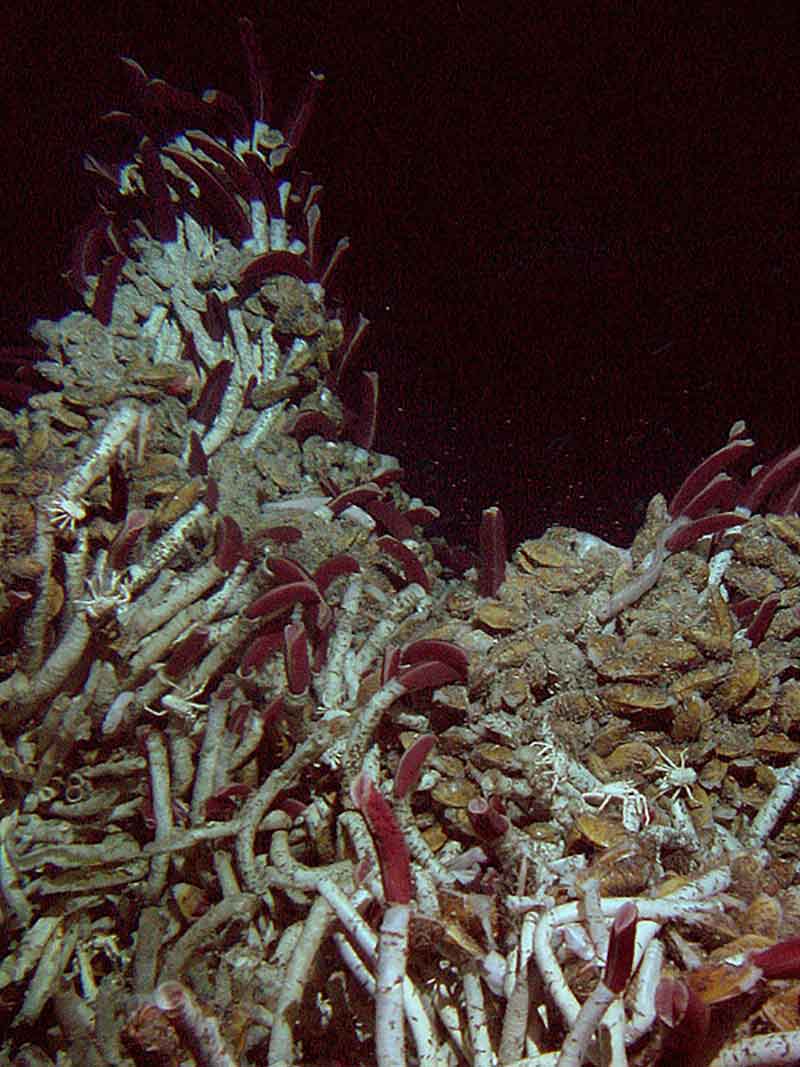This captivating photograph captures an intricate underwater scene with a nearly black backdrop, densely populated with an array of marine life. Dominating the composition are masses of tiny tube-like structures, which are likely deep-sea worms. These worms have white bases and maroon-red tips, reminiscent of upright standing cigarettes or matches. They start from the upper left corner and spread across the image, looping down to the bottom and over to the middle right. Interspersed among these tubes, particularly on the right-hand side, are areas of yellowish-green plants, adding to the vibrant diversity of the underwater tableau.

Upon closer inspection, the scene reveals a more detailed ecosystem: small, white crabs are scattered throughout, blending with the worm structures, and requiring a keen eye to spot each one. The landscape, which might first appear as a pile of debris or wood, teems with life that almost camouflages itself. Among the worms and crabs, some mollusks and clams are also visible, colonizing what looks like a pointed rock structure. This rock itself is almost entirely covered by the wormy tubes, but the sheer density and variety of life forms make this an enthralling snapshot of deep-sea biodiversity. Floating particulates in the dark background hint at the depths at which this complex and cluttered ecosystem thrives.